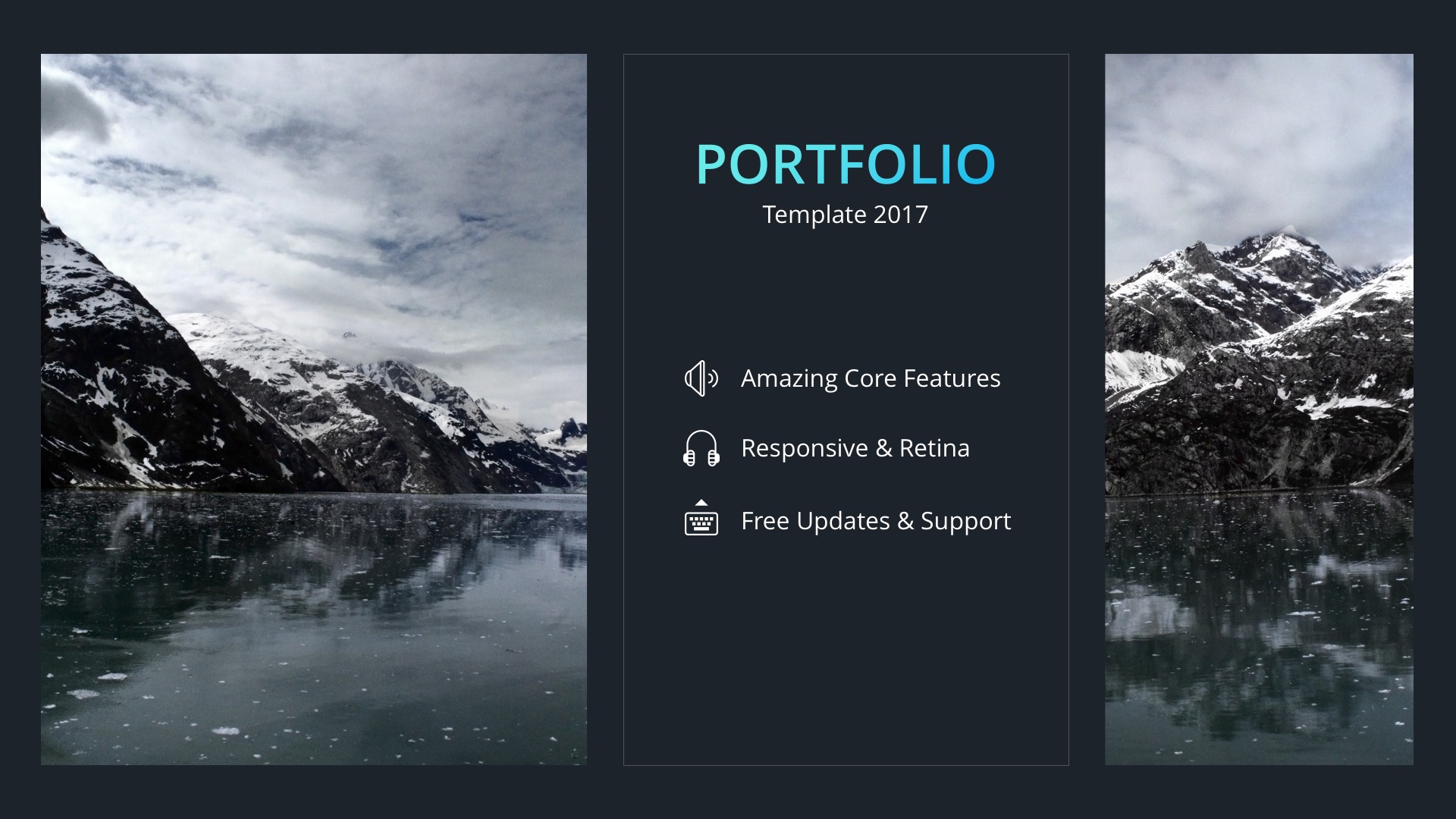This image displays a minimalistic portfolio template with a predominantly black background. The design features two photographs of equal height positioned on opposite sides, with the left image being wider than the right. In the central portion between these images, there is a black box outlined with a thin light blue border. At the top of this box, 'PORTFOLIO' is boldly written in all caps using a large light blue font. Below this, in smaller white text, is the word 'Template' followed by the year '2017'. Further down in the box, centered in three distinct rows, are the phrases 'Amazing Core Features,' 'Responsive and Retina,' and 'Free Updates and Support,' showcasing key attributes of the portfolio template.